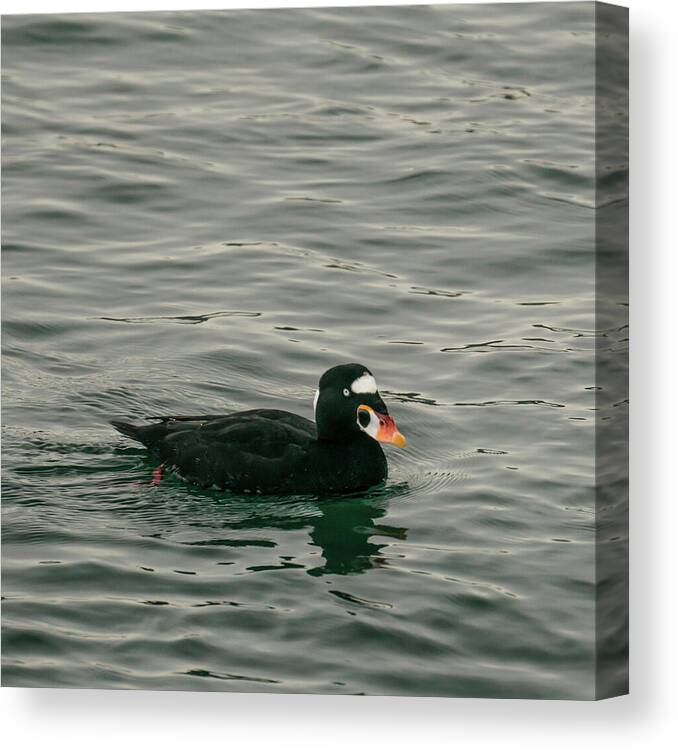The image depicts a detailed 3D-illustrated painting of a black duck swimming in dark, wavy water. The canvas, which showcases both its front and side, features a duck with a distinct white patch on its forehead and a multicolored beak with shades of orange, red, yellow, and white. The duck's eye is a striking light blue or green color, adding to its vivid appearance. The water around the duck is a mix of dark blue and gray with subtle green tones, exhibiting gentle ripples and waves, especially more disturbed behind the duck, indicating movement. On the bottom right of the canvas, the text "Fine Art America" is printed in light gray. Additionally, a slight reflection of the duck can be seen on the water's surface, enhancing the realistic and immersive quality of the artwork.